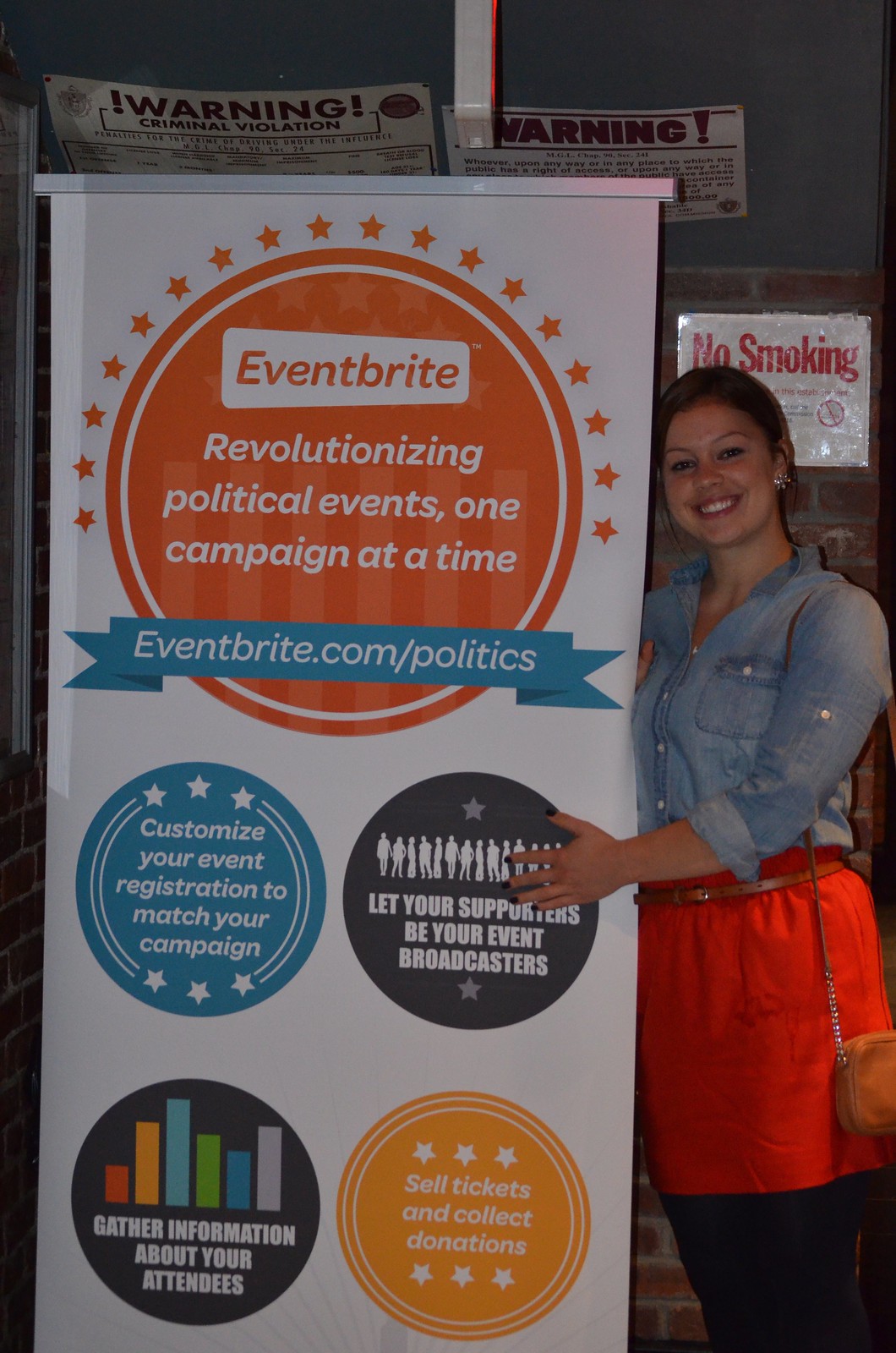This detailed photograph captures a young Caucasian woman, likely in her mid-20s, standing to the right of a prominently displayed banner. The woman has dark brown hair tied back in a ponytail and exudes an air of confidence with a broad smile, directed towards the camera. She is stylishly dressed in a denim shirt paired with a bright red skirt and leggings.

The backdrop features a partly exposed brick wall transitioning into a dark blue hue on the upper half, adding contrast to the vivid banner she is holding. The banner is primarily white and approximately four to six feet tall and two to three feet wide. Dominating the top of the banner is a large orange circle adorned with stars, containing the bold text "Everbright" and the slogan "Revolutionizing political events, one campaign at a time." Below this slogan, there is a banner that reads "everbright.com/politics."

The lower section of the banner features four distinct circles, each highlighting different functionalities:
1. A light blue circle on the left with white stars and the text "Customize your event registration to match your campaign."
2. A black circle on the right, depicting silhouettes of people and stating "Let your supporters be your event broadcasters."
3. A yellow circle showing a bar graph icon and proclaiming "Sell tickets and collect donations."
4. Another black circle to the left of the yellow one, featuring a multicolored bar graph and the words "Gather information about your attendees."

This carefully composed image not only highlights Everbright's innovative approach to political event management but also draws attention to the interactive and supportive features they offer.